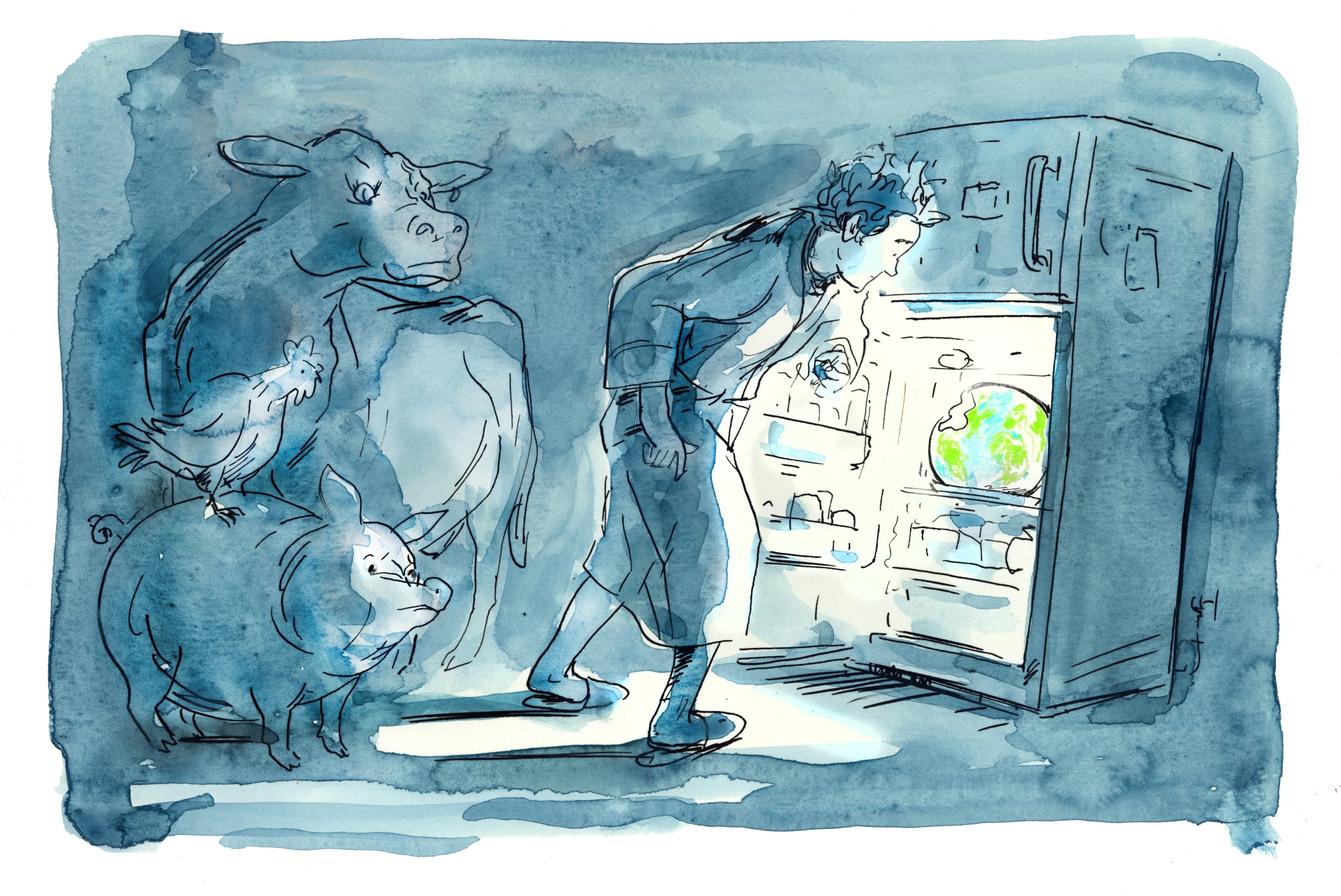In this thoughtfully illustrated watercolour cartoon set at night, we see a person opening a brightly lit refrigerator, the only part of the image devoid of the dominant blue aquarelle hues. Inside the fridge, a partially bitten planet Earth stands as the sole occupant, glowing with a stark contrast of white light against the cooler blue tones. Behind the person, a cow, pig, and chicken stand, stacked curiously with the chicken perched atop the pig, all peering into the fridge. The intricate details, from the ink pen outlines to the expressive animals, emphasize the whimsical yet poignant message that each time we eat an animal, we consume a vital part of the Earth itself.